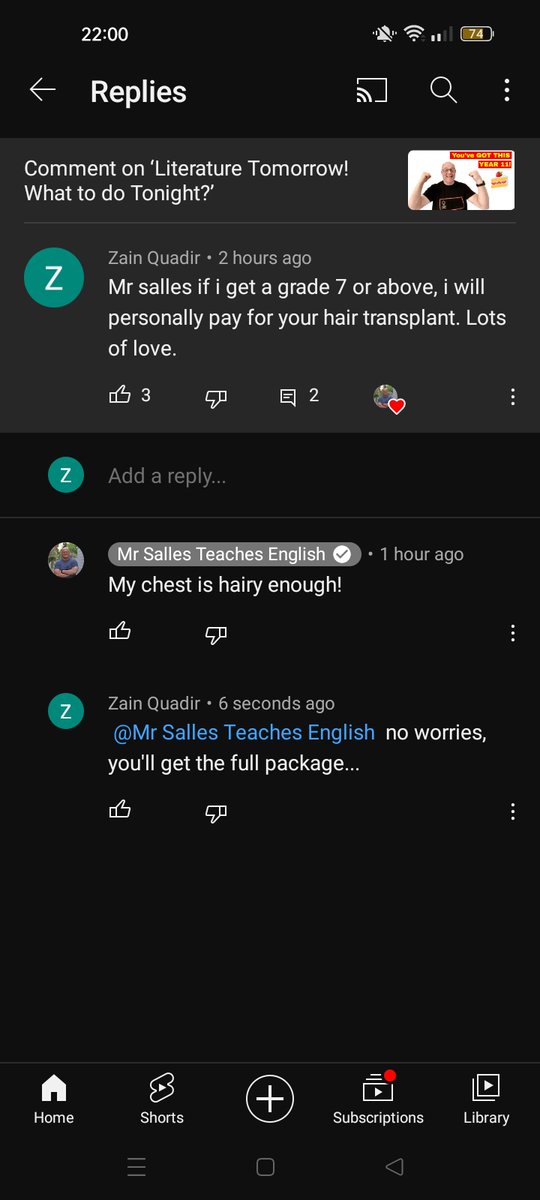This is a detailed screenshot from a mobile phone interface displaying a conversation in a message thread. At the top of the screen is the word "Replies" with a backwards-pointing arrow to its left. Below this header, there is a small strip featuring a thumbnail image of a man in a black t-shirt holding both arms up in a victory pose.

The caption under the thumbnail reads: "Comment on literature: 'Tomorrow, what to do tonight.'" Below this, a message from Zane Quadir, posted two hours ago, is visible. Zane's message reads: "Mr. Sales, if I get a grade 7 or above, I will personally pay for your hair transplant. Lots of love."

This message has received three thumbs-up reactions and appears to have been liked by the intended recipient, Mr. Sales. Following this, Mr. Sales, who is identified as an English teacher, replies humorously: "My chest is hairy enough." Zane Quadir then responds to Mr. Sales with: "No worries, you'll get the full package."

At the bottom of the screen, there are five navigation tabs.